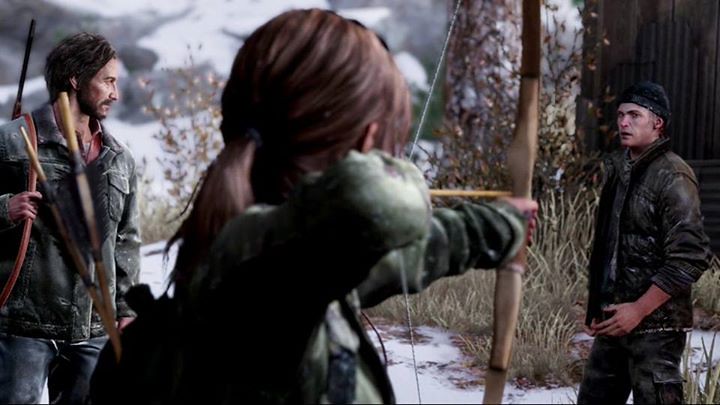The image, a screenshot from a survival video game, features a scene set in an outdoor, snowy, and wooded environment with visible hints of vegetation, including grass and leaves. The rectangular artwork captures three individuals, all appearing to be outdoors in tactical or fatigue clothing, showcasing a tense confrontation.

On the left stands a man with brown hair and facial hair. He is adorned in a grey jacket and blue pants, and he wields a gun with a shoulder strap, gripping it tightly. His expression is one of intense focus, directed towards the man on the right. 

In the center of the scene, with her back to the viewer, is a woman wielding a bow and arrow. She is actively drawing the bow, aiming it towards the man on the right. Her presence and stance indicate she is a critical figure in the confrontation.

The man on the right, a Caucasian male, dons a black beanie and looks tense as he faces the immediate threat posed by the central figure. He is positioned in front of a dark-colored building, further emphasizing the dire and survivalist theme of the setting.

In the background, a snow-covered terrain merges with bushy undergrowth and a distant hill, providing a stark and cold atmosphere that encapsulates the precariousness of the situation depicted.